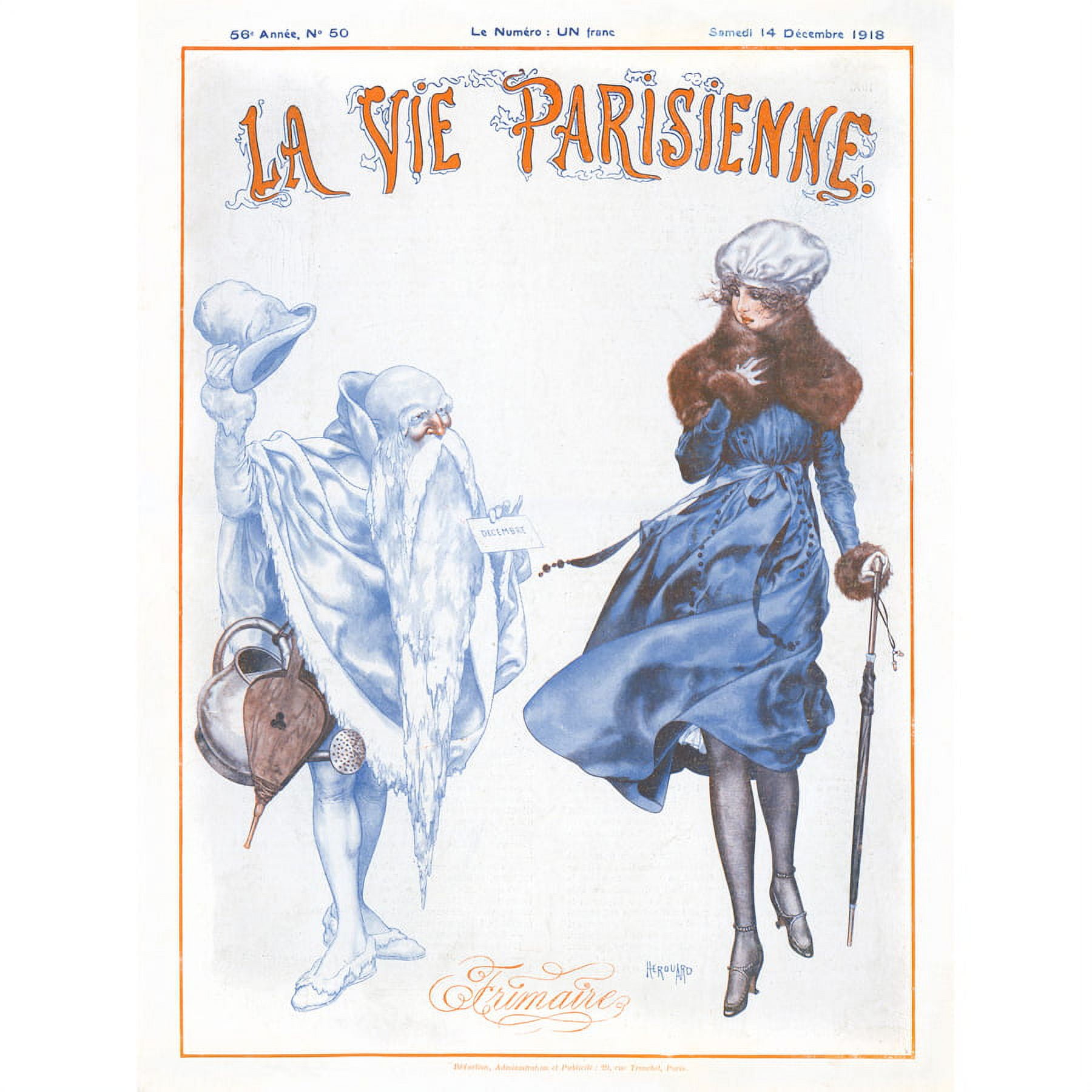This is an illustration from the cover of a December 14th, 1918 issue of the French magazine "La Vie Parisienne." The scene appears to depict a theatrical performance or a stylized encounter, likely set in a wintry, playful context. On the right, a woman stands elegantly in a blue dress paired with high heels and a fur trim around her neck and wrists. She carries an umbrella and wears a white, loose cap resembling a hairnet or a unique bonnet, containing her hair. 

On the left side of the image is an elderly figure reminiscent of Jack Frost, made of snow and ice. He sports a long white beard, a white cape, and a top hat. His features are predominantly white, except for his nose, which is pinkish-tan. The man is accessorized with a bellows and a watering can hooked to his belt, and he holds up a sign marked December. The title text at the top of the image is in French, furnishing the vintage feel and context. The artist of this intricate and whimsical scene appears to be Harard.